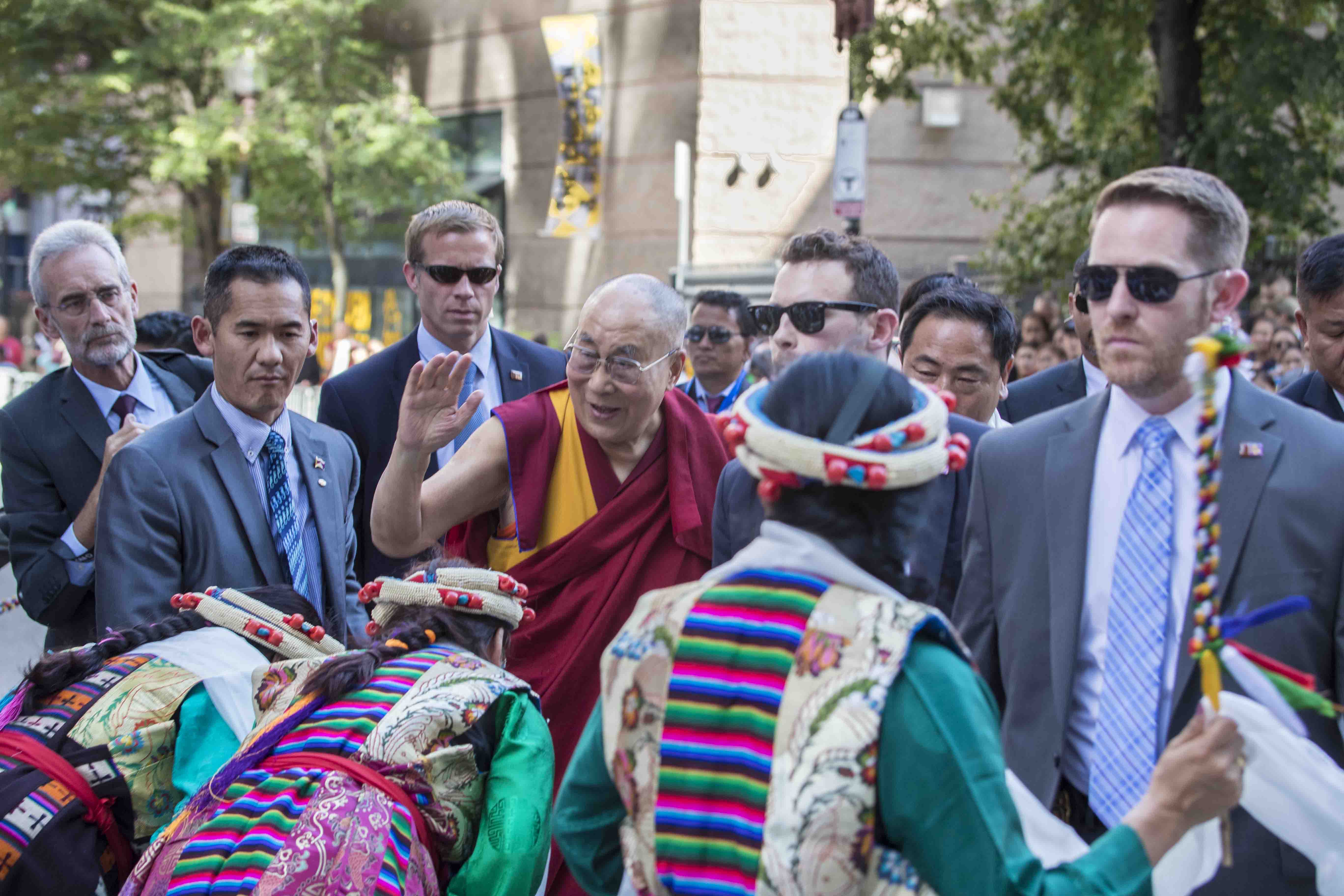In this vibrant photograph, the Dalai Lama is making a significant visit to a location in either Europe or the United States. The scene captures a group of people in traditional Tibetan clothing bowing reverently towards the Dalai Lama, expressing deep respect and admiration. Surrounding him is a contingent of security personnel, some wearing sunglasses to shield their eyes from the bright sunlight, ensuring his protection. Additional individuals, without sunglasses, are seen accompanying him as well. The day is notably sunny, with sunlight illuminating a building in the background and highlighting two large trees that add a touch of natural beauty to the scene. The Dalai Lama, radiating warmth and joy, is seen waving to the gathered crowd. His smile and the twinkle in his eyes are emphasized by his glasses. He is dressed in a traditional red and yellow Buddhist Tibetan robe, which stands out brightly against the vivid setting. This photograph encapsulates a moment of cultural richness, reverence, and the Dalai Lama's enduring charisma.